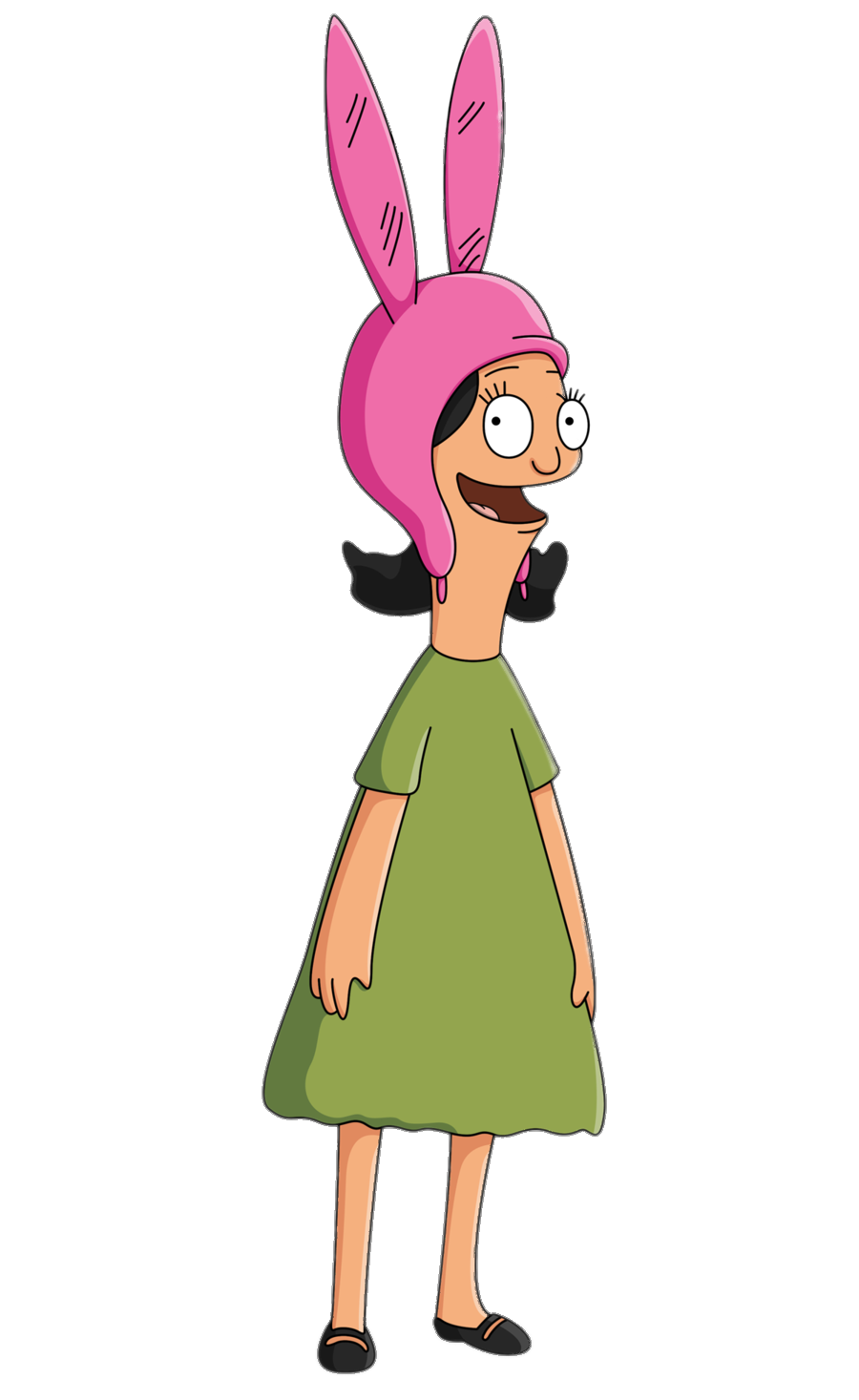The image showcases a character from the animated show Bob's Burgers, identified as Louise Belcher. She is depicted as a young girl with light skin and short black hair that flares out on either side of her head. She wears her iconic pink hood, adorned with large pink bunny ears, which snugly fits around her head and has small strings hanging from the bottom. Louise's eyes are large, wide, and white, with tiny black eyelashes, giving her an expressive look. Her mouth is open in a slight smile. She sports a green, triangular dress that reaches her knees and has short sleeves and a round collar. On her feet, she wears black shoes with a small slit on top, showing a simple yet distinctive style. In the image, Louise is angled slightly towards the bottom right corner but gazes directly at the viewer, her arms hanging naturally at her sides. The background is completely white, making her appear to float in an empty void.